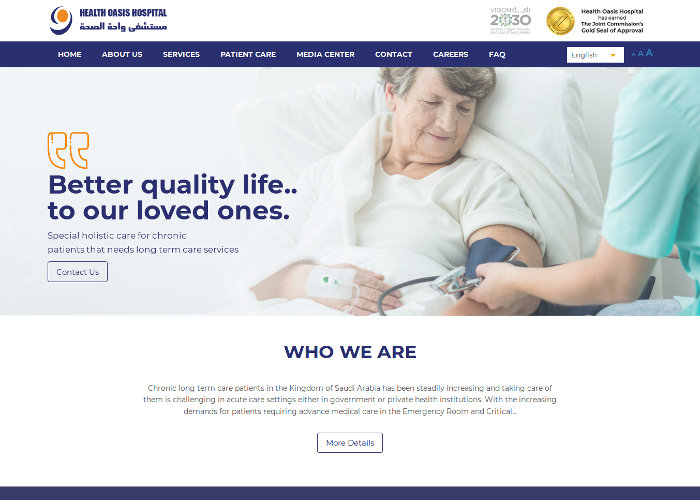The image depicts a section of a web page featuring a photograph of an elderly patient lying in a hospital bed, clad in a white hospital gown and resting on white sheets. A nurse, identifiable by her light green scrubs, is captured in profile as she measures the patient's blood pressure. A catheter is visibly connected to the patient's right hand. On the left side of the image, a large text section reads, "Better quality life to our loved ones," written in bold blue font with two orange quotation marks framing it. At the top left corner of the web page, the name "Health Oasis Hospital" is displayed in blue next to an orange circle and blue logo. Beneath this, there is an inscription in the Arabic language.